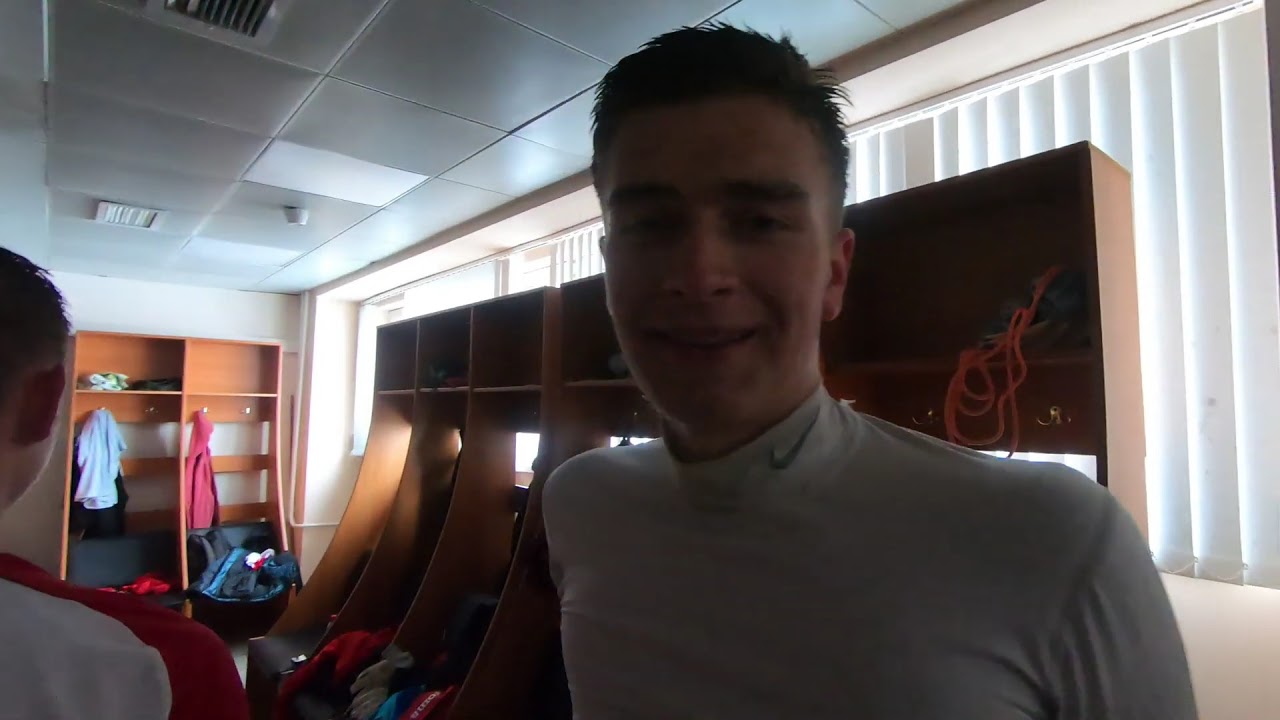This photograph captures a vibrant, sunlit locker room scene centered around a young, probably Caucasian man in his early twenties. He's sporting a white mock turtleneck shirt prominently featuring a gray Nike swoosh logo at the collar. His dark brown hair and bushy eyebrows are noticeable as he smiles at the camera. The image reveals the locker room's interior with brown wooden cubicles equipped with hooks and benches, filled with an array of colorful clothing, including pink and blue garments. To the left of the man, there is another individual in a red and white shirt, partially visible from behind. The background includes more cubicles and shelves, with white window blinds allowing sunlight to filter in, along with glimpses of the white ceiling with vents and additional storage spaces filled with hanging clothes. An orange rope can also be spotted over the man's right shoulder, adding to the detailed setting of the room.